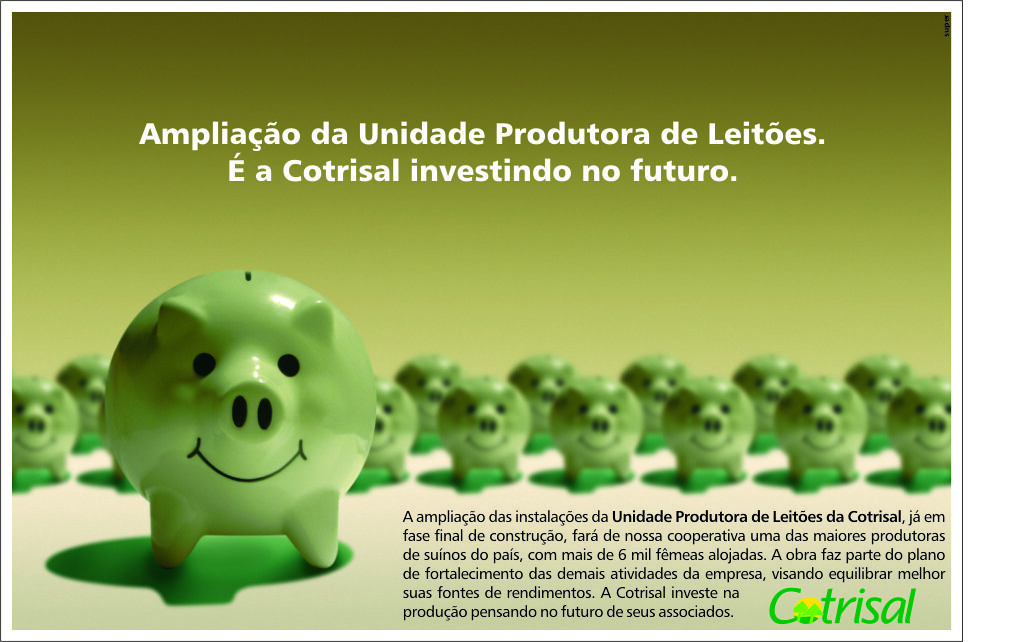The advertisement features a lime-green themed image promoting savings with Cotrisal Bank. Set against a gradient background blending green, cream, and gray hues, the focal point is a line of around 15 to 20 small, green piggy banks, each with distinct black eyes, snouts, and smiles, all facing forward. The largest piggy bank sits prominently on the left, closest to the camera. The pigs have slits on their tops, emphasizing the savings theme. Spanish text in white and black adorns the top, conveying the main message. A detailed paragraph in black text is placed towards the bottom right corner above green Cotrisal Bank branding, emphasizing the investment and future-oriented ethos of the bank. The piggy banks add a cute and engaging touch to the advertisement.